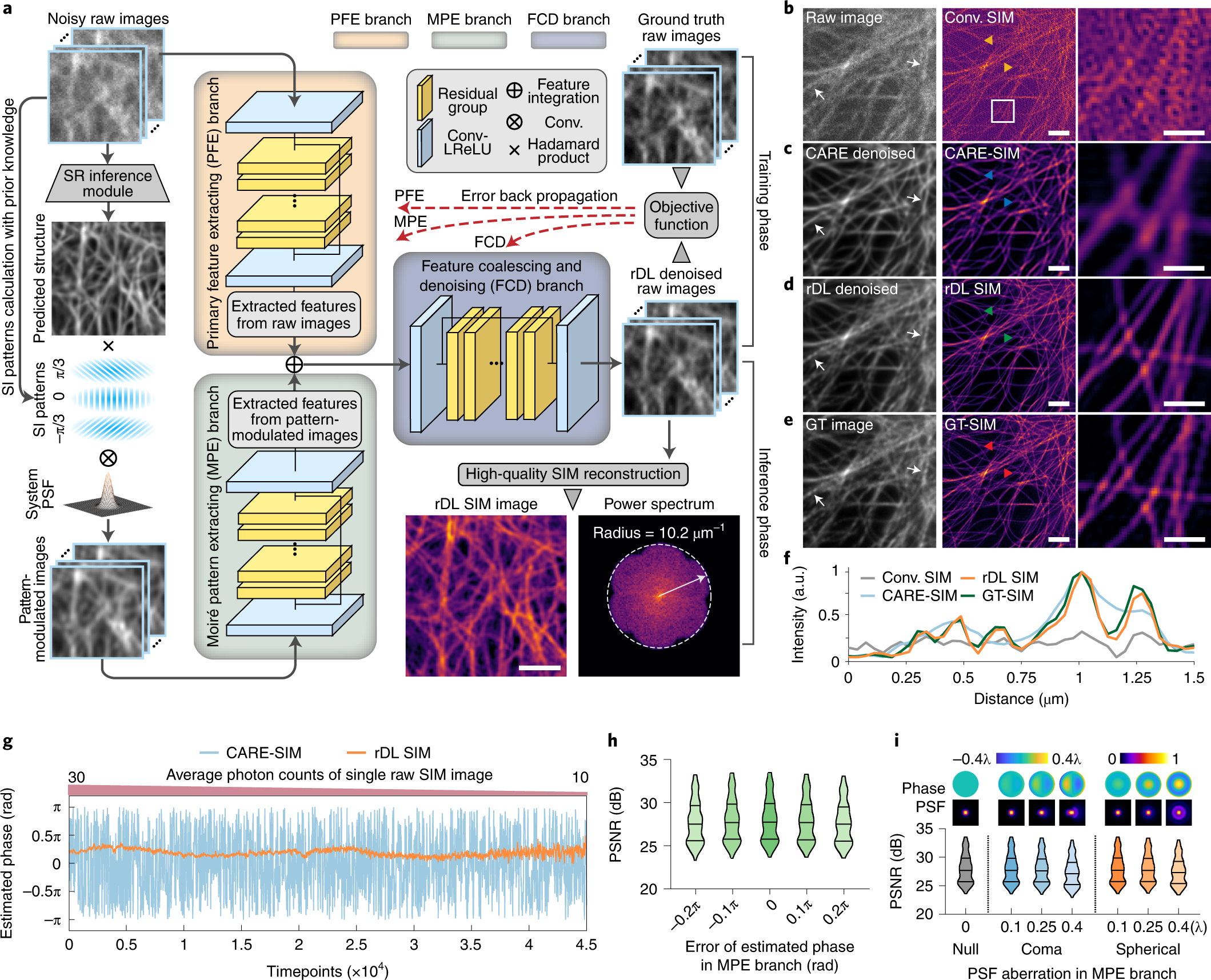The image is a detailed scientific illustration that combines multiple graphical representations and data sets concerning sim images and their analysis. The layout features nine labeled sections (A, B, C, D, E, F, G, H, I). Dominating the top two-thirds and left two-thirds of the image is section A, which highlights new studies available on Prolific and details about noisy raw images, their inference module, PFE branch, and MPE branch, including terms like "ground truth raw images" and "SR in inference module."

On the right third of the image, sections B through F feature twelve grayscale and purple images, segmented into a 4x3 grid, depicting various visual data and filters related to sim image discernment. Below these images, a graph with green, gray, and orange lines provides an analysis of distance and intensity metrics. 

At the bottom, sections G, H, and I present three different charts: G illustrates the average photon counts of single raw sim images; H shows the error distribution of the estimated phase within the MPE branch; and I details PSF aberration and the operations of the MPE branch, offering a comprehensive view of the statistical and graphical evaluations pertinent to the study.